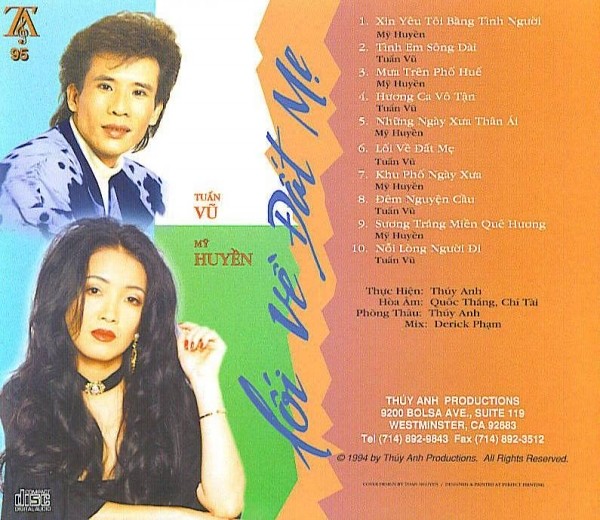The album cover features an advertisement for two Vietnamese singers, Tuan Vu and Mai Huyen, with a prominent, visually striking design. The upper half of the poster displays a photograph of Tuan Vu, an Asian man clothed in a blue outfit, looking directly at the camera. Below him is an image of Mai Huyen, an Asian woman with long, black, center-parted hair that obscures her attire, though she wears a necklace and a bracelet. 

The background features a blend of vibrant colors, including yellow, orange, and pink, creating a dynamic and eye-catching effect. To the right, a vertical list of ten songs is displayed, each accompanied by its respective singer in a foreign language, prominently showcased in white and black text respectively. The songs listed are: 
1. "XINYEUTOIBANGTINHNGUOI" by Mai Huyen
2. "TINMSONGDUWAY" by Tuan Vu
3. "MONTRENINDOWAY" by Mai Huyen
4. "WONGKAVOTAN" by Tuan Vu
5. "NUNGIUNGTIAY" by Mai Huyen
6. "LOIVEDAMAY" by Tuan Vu
7. "KUFONGIZUN" by Mai Huyen
8. "DEMNUGUENCHU" by Tuan Vu
9. "SUONGTRANGMIENQUAYUAN" by Mai Huyen
10. "NUNGGAYD" by Tuan Vu

The bottom portion lists contributors to the album including Thuc Yen, Thu An, Hoa An, Quoc Bang, Chi Tai, Phuong Tai, and Derek Pham. The production details include "Thu An Productions, 9200 Bolsa Avenue Suite 119, Westminster, CA 92683," with the contact telephone number 714-892-9843 and fax number 714-892-3512. The album was released in 1994, as indicated by the copyright notice: "© 1994 by Thu An Productions, all rights reserved."

Overall, the poster features a harmonious mix of colors and detailed elements that highlight both the artists and their music.